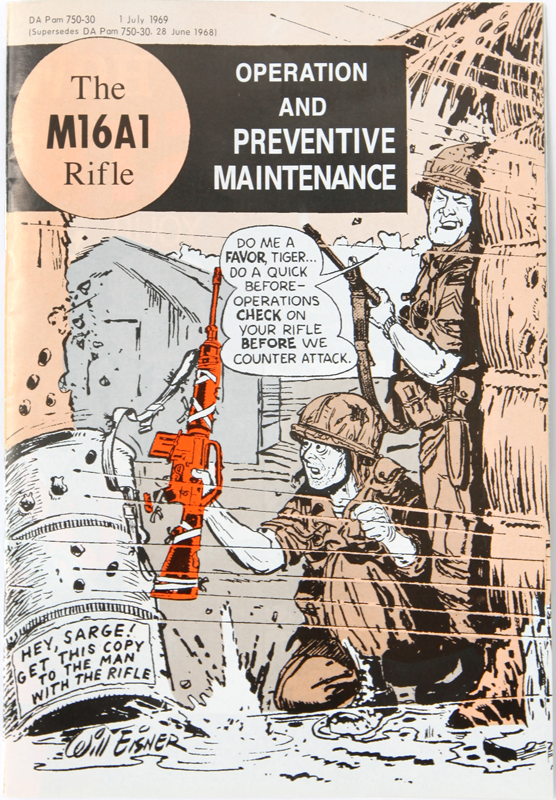The image is a detailed comic book page titled "Operation and Preventive Maintenance" prominently displayed at the top. On the left side of the title, it says "M16A1 Rifle" in white, capital letters within a pink circle. The artwork is predominantly in a light beige color. Central to the image are two soldiers wearing brown uniforms and helmets. One soldier is standing on the right side, holding a brown rifle, and the other is kneeling on the ground to the left, clutching a distinctive bright orange rifle, which appears patched and bandaged. The standing soldier addresses the other with a conversation bubble saying, "Do me a favor, Tiger. Do a quick before operations check on your rifle before we counterattack." To the left side of the scene, there's a tall barrel. At the bottom left of the page, handwritten in a casual font, it reads, "Hey, Sarge, get this copy to the man with the rifle. Will Eisner." The setting seemingly includes a grass hut in the background, adding to the detailed narrative of the scene.